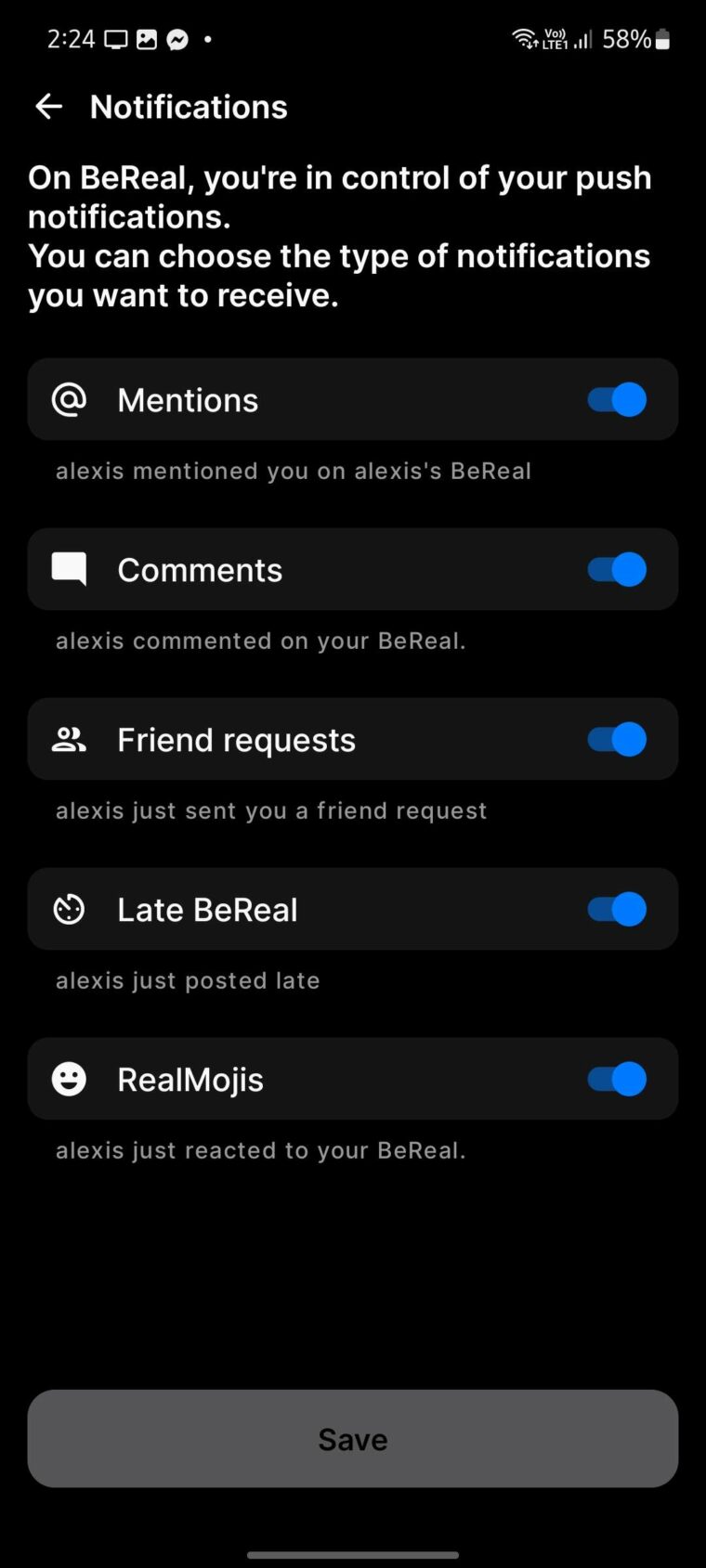The image depicts a device screen with a black background. In the top left corner, the number "224" is displayed, followed by a monitor icon, a picture icon, and a messenger icon, all in white. On the top right corner, there are icons for Wi-Fi, cellular network, and battery, which shows 58% remaining charge.

Below these icons, a white arrow points to the left, and the text "Notifications" is displayed next to it. The main content below this header reads: "On BeReal, you're in control of your push notifications. You can choose the type of notifications you want to receive."

The interface contains five sections for different types of notifications:

1. **Mentions**: Displayed with an "@" symbol, it states, "Alexis mentioned you on Alexis’ BeReal."
2. **Comments**: Shows that "Alexa commented on your BeReal."
3. **Friend Requests**: This section is labeled but not described in the provided text.

Each section is clearly divided, offering users a streamlined and user-friendly notification management system.